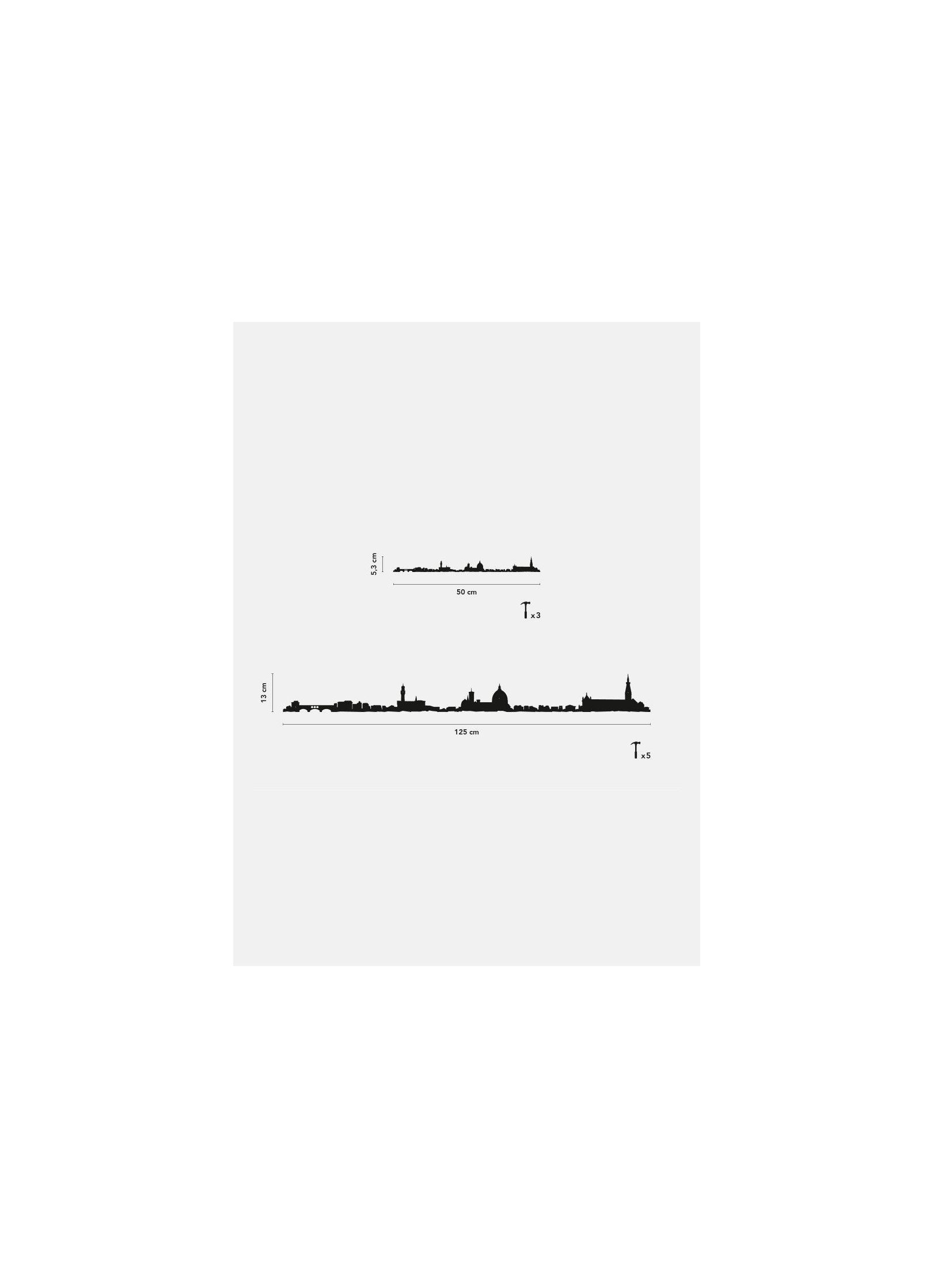The image features a minimalist design with black silhouettes of a city skyline on a gray background. At the top, a smaller skyline illustration is centered, showcasing various city buildings, some taller while others exhibit rounded features. Directly below it, on the right side, is an image of a hammer. Underneath both, another larger version of the same skyline is depicted, aligned centrally.

Both skyline illustrations are accompanied by labeled axes. On the y-axis, one reads "5.3 centimeters" and the other "13 centimeters", while the x-axis labels show "50 centimeters" and "125 centimeters". Beside the hammer, there are two sets of text, one reading "times 3" and the other "times 5". The overall style conveys a cityscape at different scales, with clear black outlines standing out against the subtle gray backdrop.